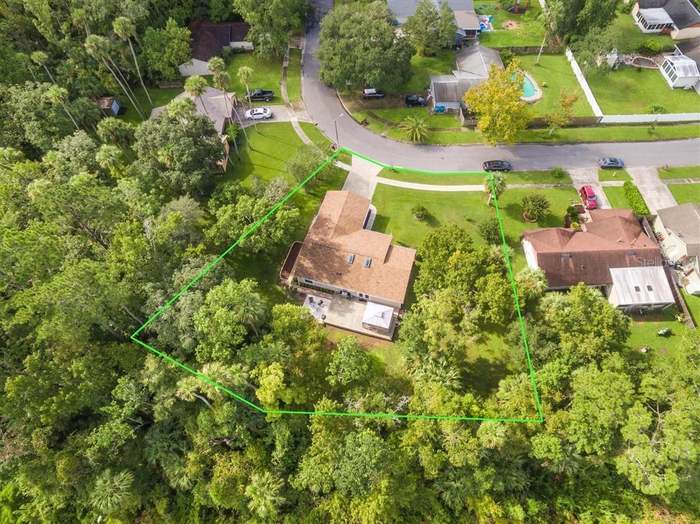This detailed aerial real estate photo showcases a neighborhood segment, highlighting a specific property with a green overlay indicating its boundaries. The featured home, positioned centrally, is surrounded by abundant tree canopies, creating a verdant landscape on the lower and left sides of the image. The house, marked by a brown roof, boasts a long concrete driveway leading to a curved road. To the upper left, another home, nestled amidst palm and tall trees, has a white car in its driveway. On the right, the top of an adjacent house with a red SUV and another car parked on the corner are visible. Across the street to the upper right, a side view reveals a house with a pool in the backyard. Overall, the photo emphasizes the lot lines and greenery, illustrating the property's expanse and its context within the neighborhood.